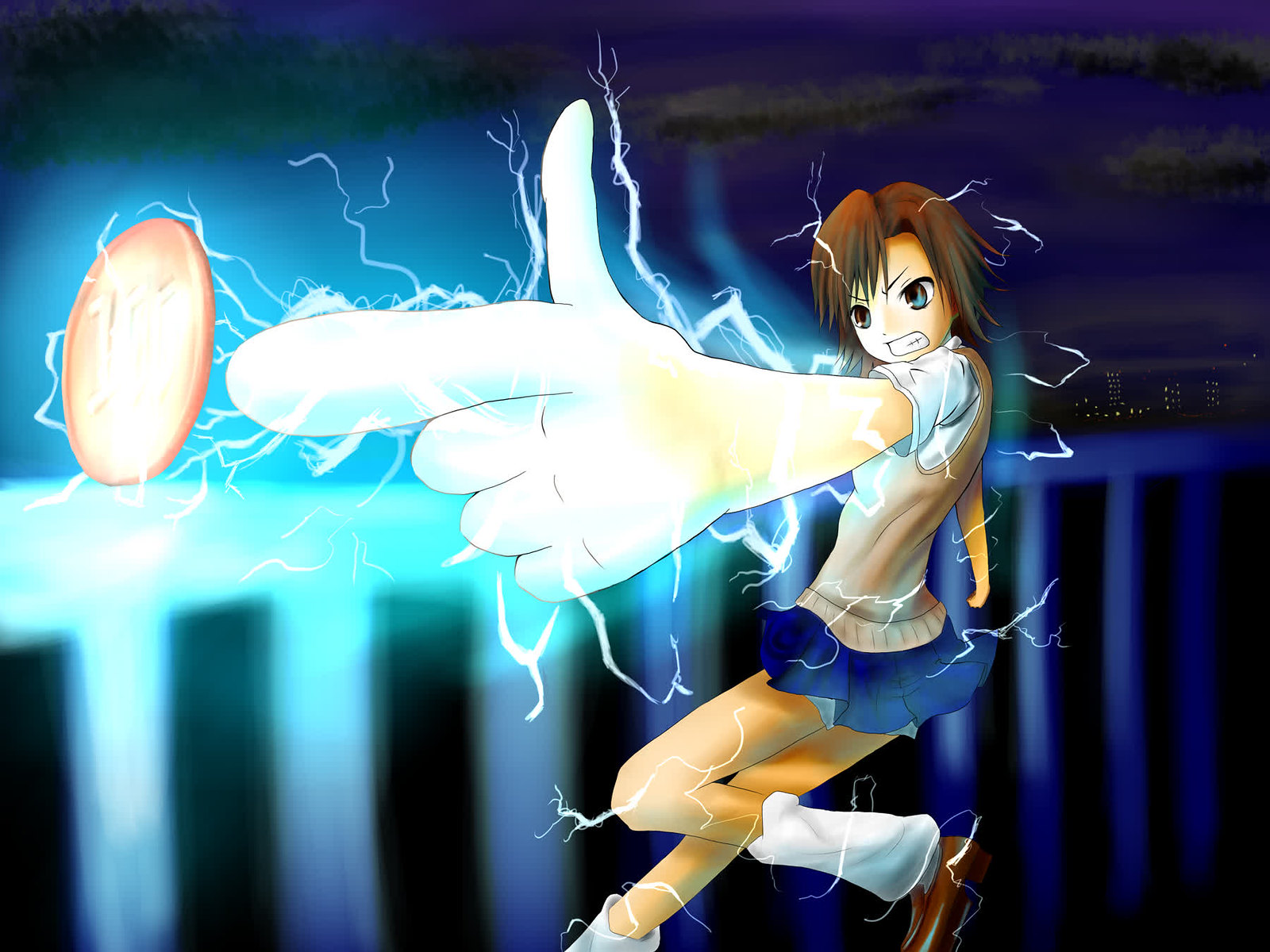In this digitally-rendered, cartoonish image, a young girl with light brown hair and intense blue eyes is depicted in a dramatic nocturnal setting. She stands in front of a blue railing with her arm stretched out, pointing like a gun toward a glowing yellow disc marked with the number one. Her other arm is flung behind her, and she is surrounded by crackling electrical lightning bolts, suggesting an aura of power. The girl wears a short-sleeved white shirt beneath a beige sweater vest, paired with a short blue skirt, white socks, and brown shoes. The backdrop features a cityscape with distant lights and buildings under a dark, cloudy sky tinted with deep blue hues, enhancing the image's atmospheric tension. The composition has a vertical orientation, reminiscent of a screenshot from a video game, and captures her energetic stance seemingly mid-action, contributing to the dynamic and engaging visual narrative.